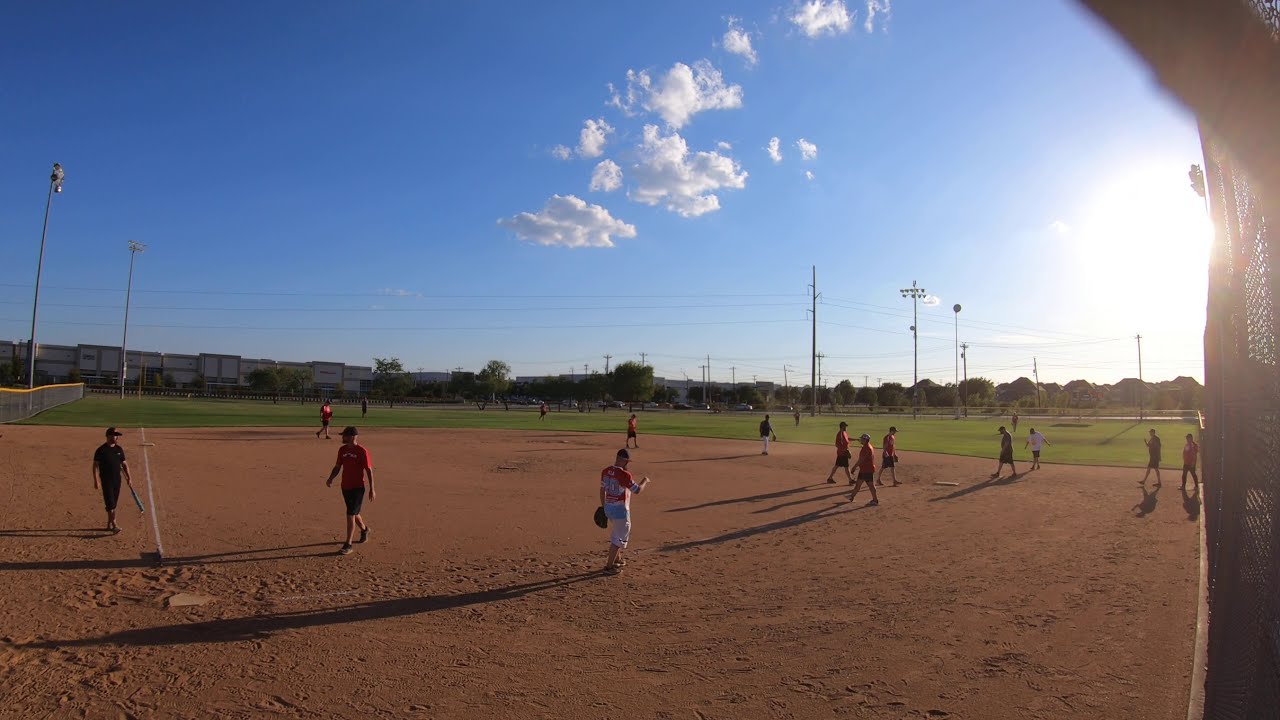The image captures a lively scene set on a normal dirt baseball diamond at a park, with a grassy outfield extending into the distance. The photo is taken from the perspective of someone slightly to the left of a dark, partially visible gate. In the foreground, several adults in red jerseys meander aimlessly around the diamond, not adhering to typical game positions. One player, equipped with a glove on his left hand, is gesturing with his right arm as if ready to throw a ball, while others seem less focused, possibly just enjoying a casual moment. The background features a mix of open green fields with no bleachers, silhouettes of distant buildings, clusters of trees, and a web of power lines cutting across the sky. The weather is sunny, with a bright blue sky peppered with a few white clouds, and field lights standing unused, casting gentle shadows on a picturesque day.